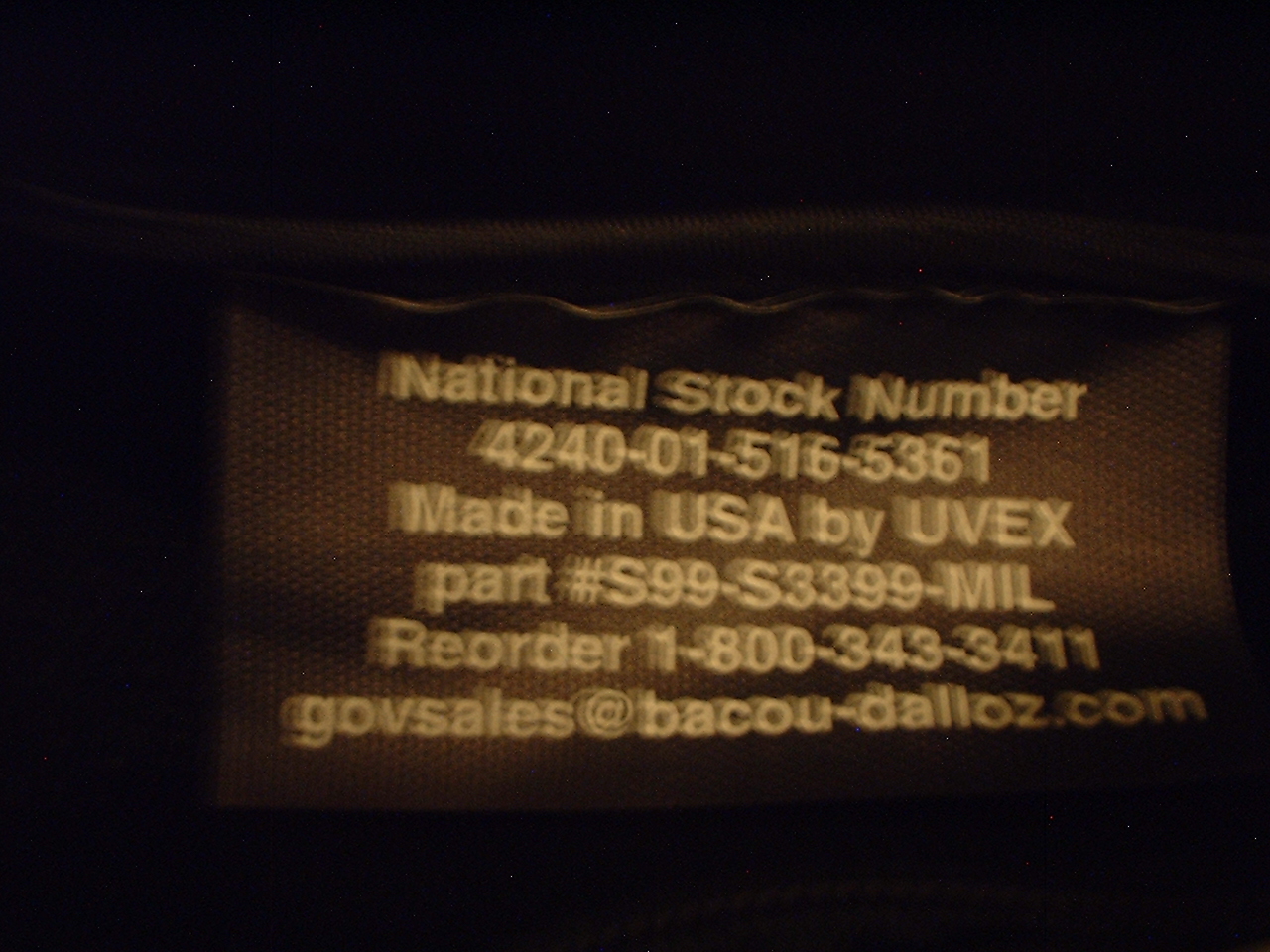This is an indoor color photograph, capturing a close-up image of a tag on a piece of clothing or packaging. The tag features white text on a dark brown, blackish background. The label reads: "National Stock Number 4240-01-516-5361. Made in USA by UVEX. Part Number S99-S3399-MIL. Reorder: 1-800-343-3411. Email: govsales@bacou-dalloz.com." The edges of the image are black, and while the photograph is somewhat out of focus, the label remains legible.